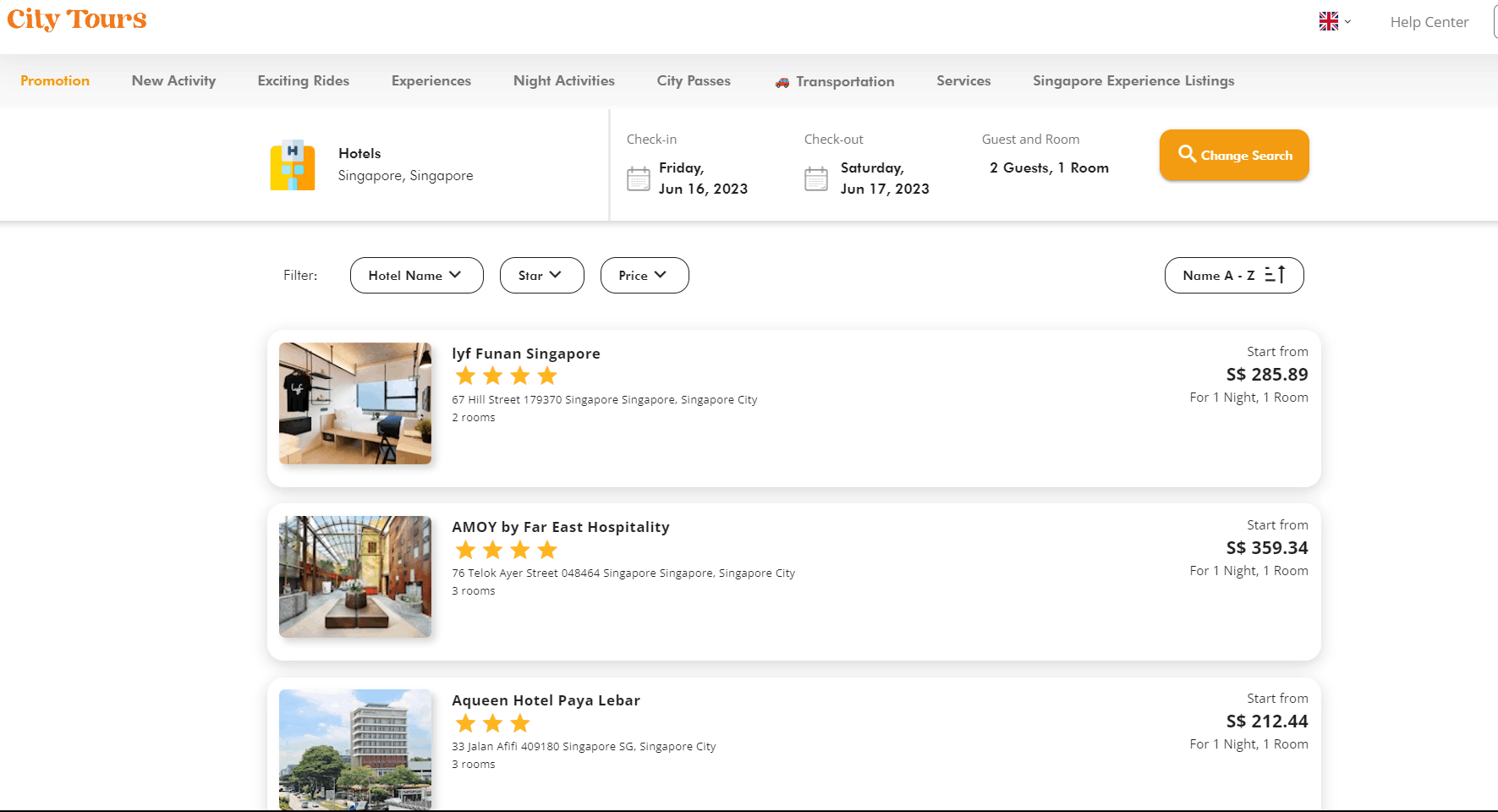The image depicts a search interface on a website dedicated to city tours, set against a predominantly white background with a slim, light gray border at the top, about half an inch in thickness. In the upper left corner, the text "City Tours" is prominently displayed in orange. On the upper right, there is a small square featuring a red plus sign, positioned next to a black "Help Center" label.

Beneath the white header area and within the light gray border, there is a horizontal menu of clickable options. The first tab, highlighted in orange, reads "Promotion." Following it to the right, in sequence, are tabs labeled "New Activity," "Exciting Rides," "Experiences," "Night Activities," "City Passes," "Transportation" (with a car icon to its left), "Services," "Singapore," and "Experiencing Listings."

Directly below the "Exciting Rides" tab, there is a small orange icon resembling a building, featuring a white square with a black letter "H" at the top, two small light blue windows, and a large light blue door below. Beside this icon, the word "Hotels" is highlighted in bold text, with "Singapore, Singapore" specified underneath.

To the right of the hotel icon, the interface provides a section for Check-In Information, Check-Out Information, Guest Room details, and the number of rooms, followed by an orange "Change Search" tab featuring a search icon.

Below this section, a thin black border separates the upper menu from filter options. The filter area includes three white tabs with black borders labeled "Hotel Name," "Star," and "Price." To the right of these filters, there is another tab labeled "Name A-C."

Beneath the filter options, the results for three hotels are displayed. Each listing includes a picture on the left, the hotel's name, its star rating, and on the right side, details such as the number of rooms, the number of nights, and the total cost.